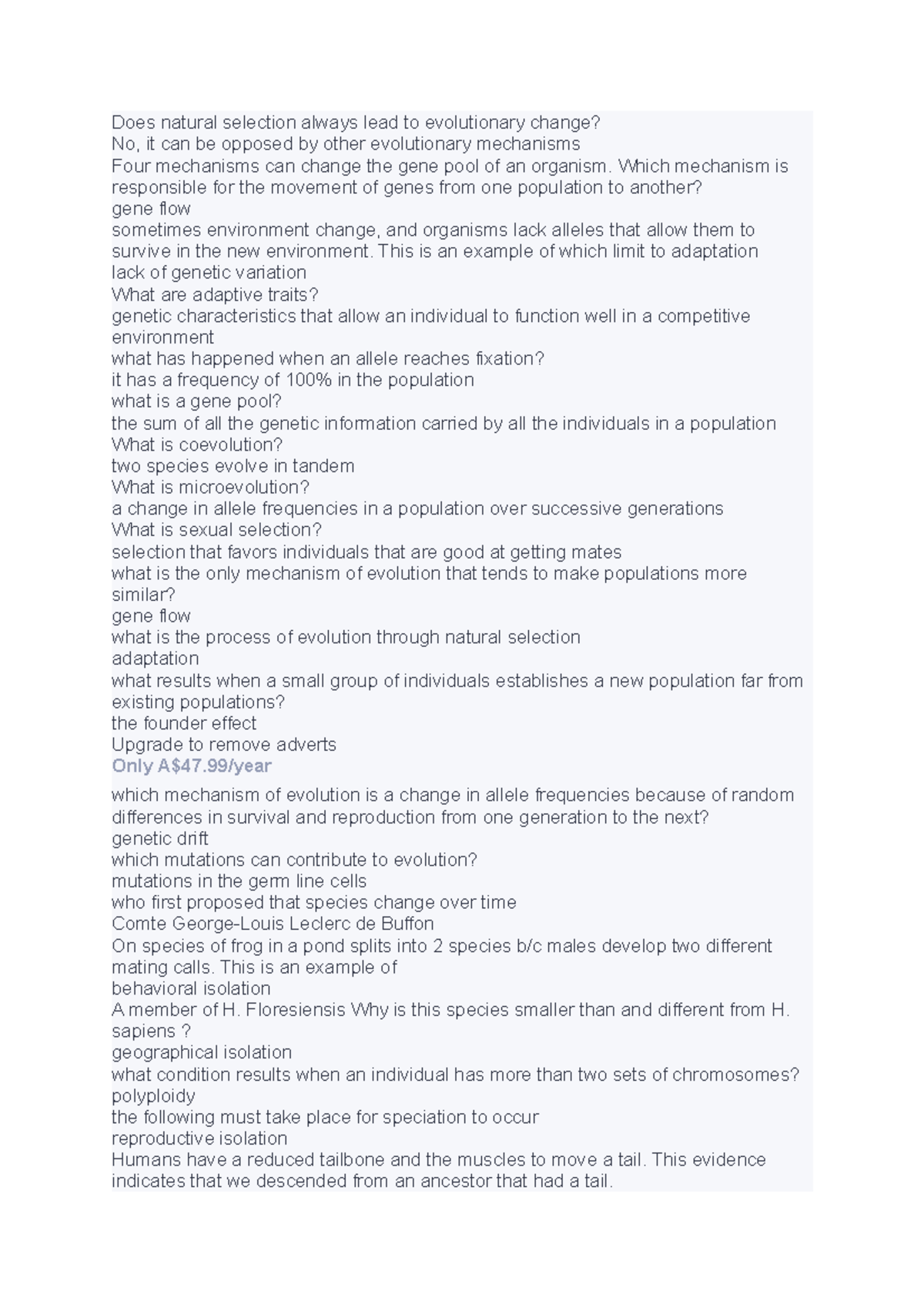This image features a passage from an educational app or website, displayed on a clean white background with black text. The primary heading in bold reads, "Does natural selection always lead to evolutionary change?" followed by the succinct answer, "No, it can be opposed by evolutionary mechanisms." Below this, the image presents an array of additional questions related to evolutionary biology, including: "What are adaptive traits?", "What has happened when an allele reaches fixation?", "What is coevolution?", "What is microevolution?", "What is sexual selection?", and "What is the process of evolution through natural selection and adaptation?" Each question is accompanied by a brief, one-sentence answer. Additionally, there is a note indicating that users can upgrade to remove advertisements for $47.99 per year. Further questions related to the topic are listed beneath this section, continuing the educational exploration of evolution.